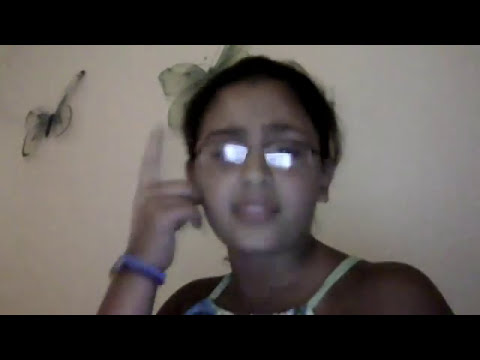The image depicts a close-up, somewhat pixelated and blurry screenshot from what appears to be a YouTube video. The focal point is a young South Asian woman with dark skin and short black hair, which is likely styled in a bun or ponytail that is out of view. She has glasses, which reflect a bright white light, obscuring her eyes. She is facing forward, smiling slightly with her mouth just barely open, showing the top row of her teeth. The woman is wearing a spaghetti strap tank shirt with pale green straps, and a light purple bracelet or watch adorns her right wrist. With her right hand, decorated with the bracelet or watch, she points upward to a delicate bow or butterfly hair accessory on the left side of her head. In the background, on what seems to be a light-colored wall, there are two artistic-style butterfly decorations positioned to the left and above her head. The overall image quality suggests it was taken with a low-resolution webcam, contributing to its dark, grainy, and pixelated appearance. The image frame is bordered thinly at the top and bottom.